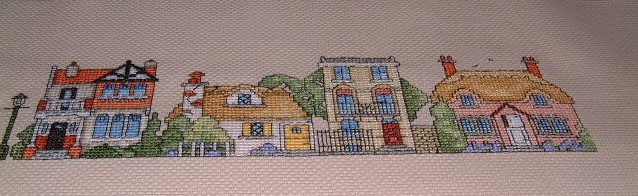The image depicts a detailed and colorful cross-stitch art piece of a quaint street scene, showcasing a series of charming houses and associated elements. 

Starting on the far left, there's a black lamppost, intricately stitched to mimic wrought iron. To its right stands a picturesque two-story white house with a dark brown door and numerous windows, characterized by its lovely brickwork and chimney on the left. Surrounding this house is lush greenery and shrubbery.

Next is a white cottage-style house, adorned with charming yellow shutters and a matching yellow front door. This cottage also features a chimney with lines that suggest creeping ivy, and quaint crisscross hatching on the windows.

Further right, a large tree marks the presence of a substantial three-story townhouse, notable for its off-white color and red door, surrounded by a gate that adds to its classic townhome feel. The townhouse has five windows on its front and additional greenery, suggesting a thoughtfully kept garden area.

Closing the scene is a pink, two-story cottage with two symmetrical chimneys and a white front door, flanked by evenly spaced windows on both floors. This house exudes balance and charm with its pastel façade.

The entire ensemble is set against the subtle backdrop of a white canvas, enhancing the vividness of the cross-stitched elements, making it both a decorative and engaging piece of art.